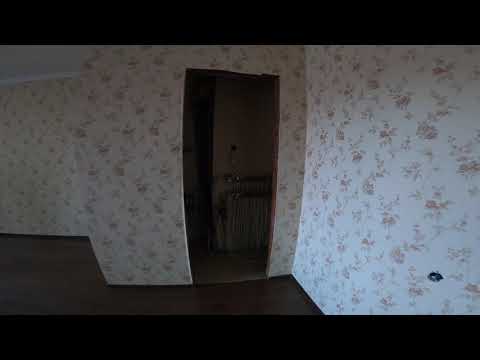The photograph captures an interior scene of an empty, older house, characterized by a dimly-lit atmosphere. Central to the image is an open doorway leading into a darker adjacent room, where parts of an old-fashioned wall radiator or furnace are partially visible against a white wall. The room features dark wood flooring, adding a touch of warmth amidst the subdued lighting. Notably, the walls are adorned with vintage wallpaper, cream in color with a delicate pattern of light pink roses, evoking a nostalgic sense that hints at decor styles from the 1970s or 1980s. The architectural layout is somewhat unconventional; the wall from the open doorway extends to a corner and bends out of sight, creating a slightly disorienting spatial perspective. This older house detail is enhanced by black horizontal lines at the top and bottom of the photograph, framing the scene in a distinctive manner.